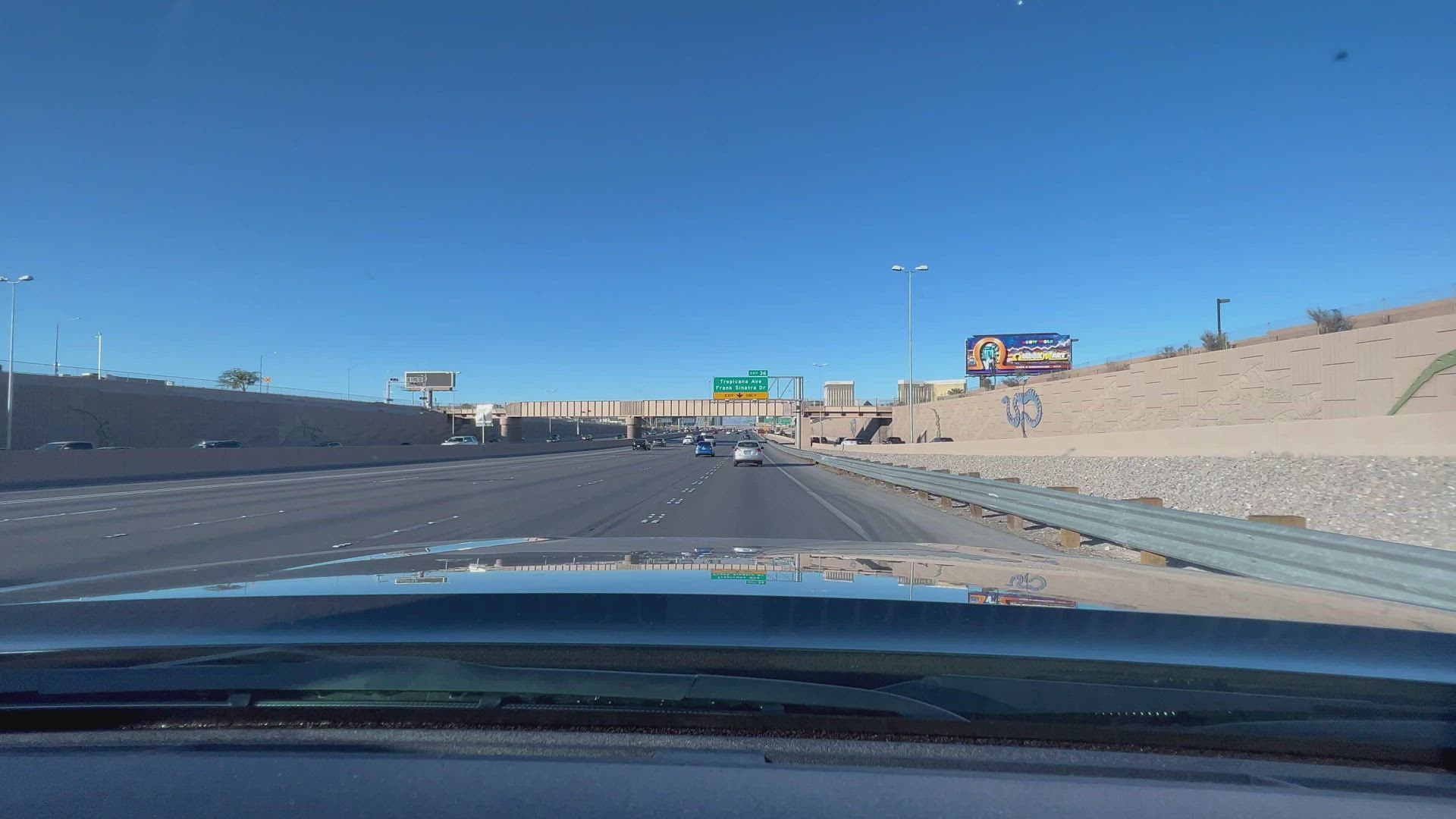This photograph captures a vibrant scene on the 215 highway in Las Vegas. In the foreground, a prominent billboard advertising Omega Mart stands out, hinting at its connection to the intriguing attractions within Area 15, an immersive art and entertainment complex. On the right side, the billboard's colorful and eclectic design makes it a focal point, attracting the attention of drivers passing by. Additionally, decorative snake sculptures add a unique touch to the roadside, contributing to the city's signature flair and creativity. The highway itself is bustling with numerous cars, reflecting the constant movement and energy typical of Las Vegas. The image beautifully encapsulates a moment of urban life in this dynamic city.